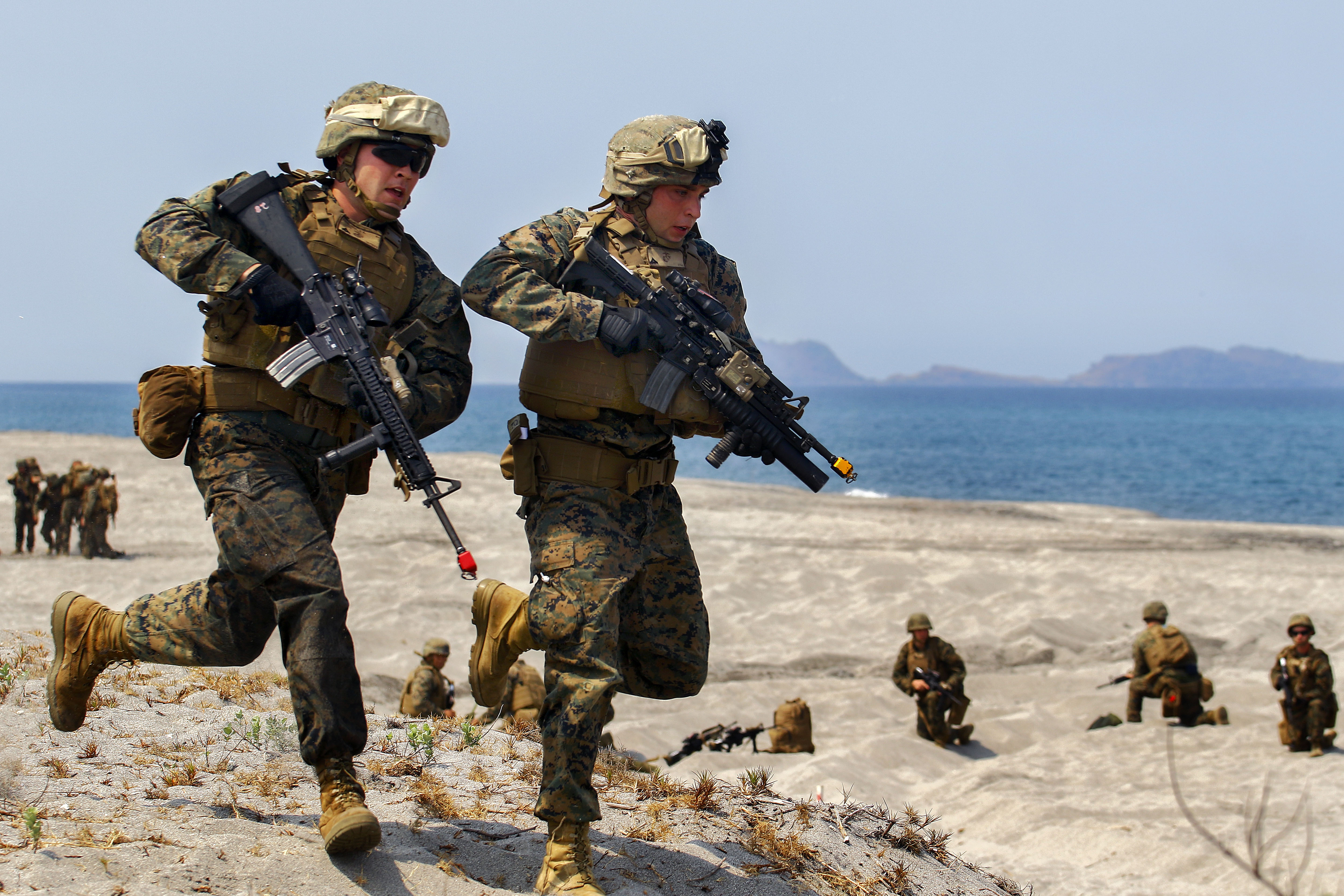The image depicts a training exercise of Soldiers or Marines on a sandy beach with the ocean and distant mountains in the background. It is a bright daytime scene, evidenced by the shadows cast by the two Soldiers or Marines in the foreground. They are fully dressed in green camouflage combat gear and beige boots, with rifles that have colored tips, indicating that they are non-operational for this drill. In the foreground, two soldiers are actively engaged, while in the middle ground, others are either kneeling, standing, or in various positions, all participating in the exercise. The clear blue sky adds to the overall bright and vivid atmosphere of the scene.